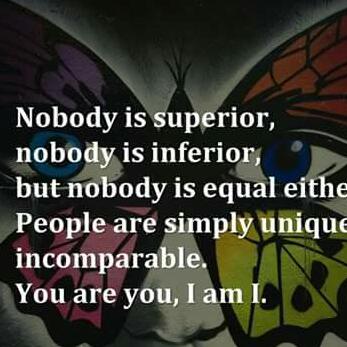The image features a visually striking poster set against a dark background, showcasing a colorful butterfly with a unique twist. Each of its four wings displays a different vibrant hue: the top left wing is purple with black accents, the bottom left wing is pink similarly detailed, the top right wing is a reddish-brown, and the bottom right wing is a yellowish-green. Intricate dots and lines embellish the wings, adding to their vividness. Interestingly, the butterfly incorporates human facial elements, with two blue eyes appearing between the upper wings, and beneath the lower wings sits the outline of a nose, subtly suggesting a face. The butterfly's body is entirely black, matching the poster's dark backdrop. Overlaying this colorful, face-like butterfly is a profound quote in white text: "Nobody is superior, nobody is inferior, but nobody is equal either. People are simply unique, incomparable. You are you, I am I." The eyes of the butterfly, seemingly gazing directly at the viewer, add a layer of depth and introspection to the artwork.